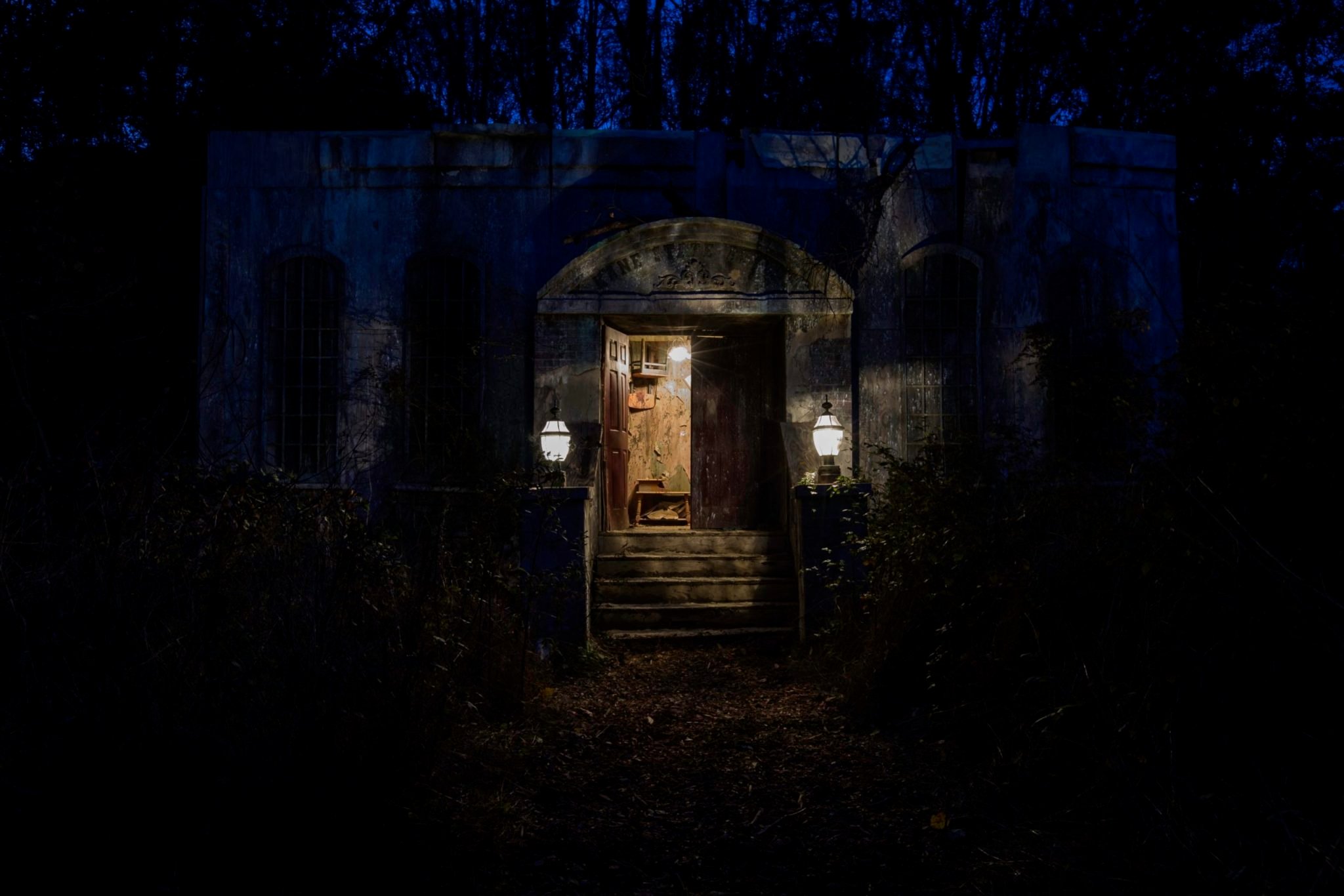This eerie nighttime scene depicts a small, abandoned concrete building that resembles a mausoleum or a large tomb, nestled in a remote forest. The building, with its brown exterior, features two tall, gated windows and an open entrance flanked by two glowing lamps. The steps leading into the mausoleum-like structure are partially illuminated, revealing a single chair hanging upside down from the ceiling inside. The environment is shrouded in darkness, with a moody atmosphere, punctuated by bluish hues peeking through black branches, and scattered brown leaves on the ground, adding to the haunting, yet oddly inviting ambiance.